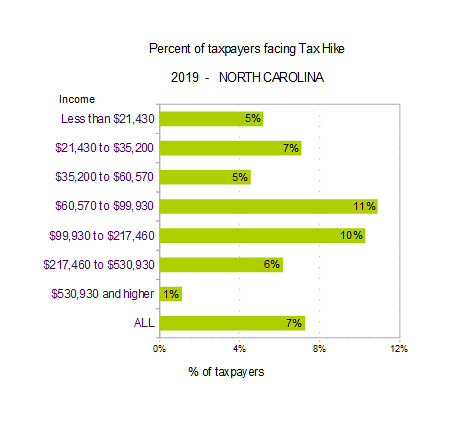The image depicts a detailed bar graph titled "Percent of Taxpayers Facing Tax Hike, 2019, North Carolina" in black ink on a white background. The graph features a column listing different income brackets in purple letters on the left side, with corresponding green bars to the right indicating percentages. 

From top to bottom, the income categories and their respective percentages are as follows:

- Less than $21,430: 5%
- $21,430 to $35,200: 7%
- $35,200 to $60,570: 5%
- $60,570 to $99,930: 11%
- $99,930 to $217,460: 10%
- $217,460 to $530,930: 6%
- $530,930 and higher: 1%
- All taxpayers: 7%

The percentages on each green bar represent the proportion of taxpayers within each income bracket who are facing a tax hike, with a final note indicating that 7% of all taxpayers are affected.